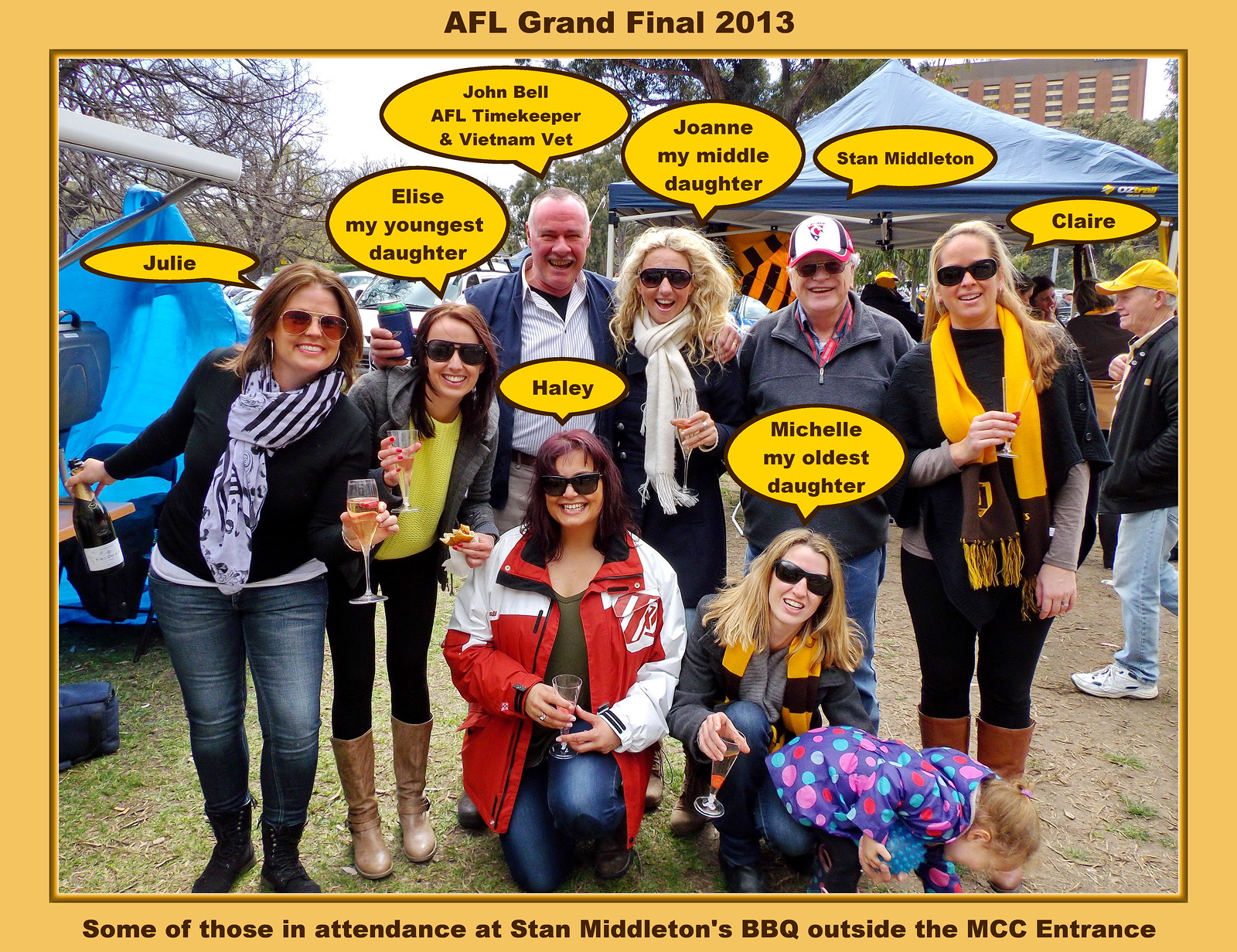In this detailed photograph taken during Stan Middleton's outdoor barbecue at the MCC entrance, we see eight people posing happily for a group photo under a bright, light brown border. At the top of the border, bold black text reads "AFL Grand Final 2013," and at the bottom, the caption states "some of those in attendance at Stan Middleton's BBQ outside the MCC entrance."

The group comprises six women and two men, all clustered closely together. The names of the people are denoted in speech bubble-style text above their heads: Julie, Elise, John Bell (an AFL timekeeper and Vietnam vet), Haley, Michelle, Joanne, Stan Middleton, and Claire. Among these individuals, two women are kneeling in front, and one of them is holding a little girl in her lap, who appears to be playing with the dirt, oblivious to the photograph.

In the background, a scenic outdoor setting unfolds with several trees, tents, and people milling about, enhancing the lively atmosphere of the barbecue. The group is enjoying themselves, and five of the women can be seen holding wine glasses, contributing to the festive mood of the gathering.